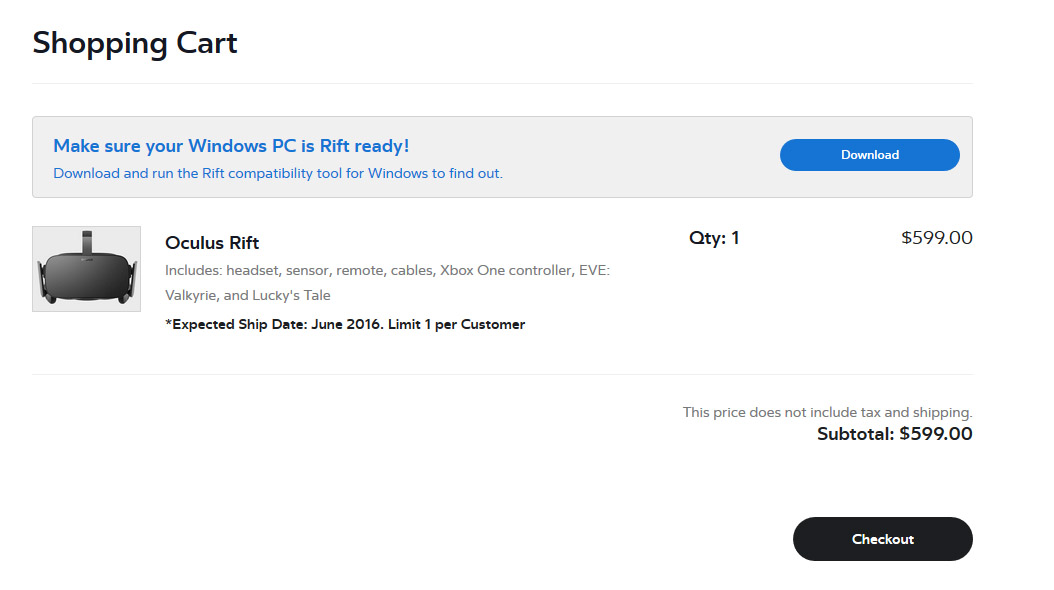This image depicts a shopping cart screen for the Oculus Rift. At the top left, the words "Shopping Cart" are displayed prominently. Directly below, a blue instructional text reads, "Make sure your Windows PC is Rift ready. Download and run the Rift compatibility tool for Windows to find out." To the right of this message, there is an oval-shaped, gray "Download" button with white lettering. This whole section is set against a gray background.

Underneath this section, the product "Oculus Rift" is detailed. On the left side, a picture of the Oculus Rift is displayed within a gray square background. To the right, a list outlines the included items: a headset, sensor, remote, cables, Xbox One controller, Eve, Valkyrie, and Lucky's Tale. Below these details, it states, "Expected ship date: June 2016, limit one per customer." Adjacent to these details, the quantity is set to one and the price is listed at $599. A note below specifies, "This price does not include tax and shipping," with a subtotal of $599.

At the very bottom, there is a black "Checkout" button with white text centered in it. The entire background of the image is white, except for the top section, which contains the gray background surrounding the compatibility instructions and download button.